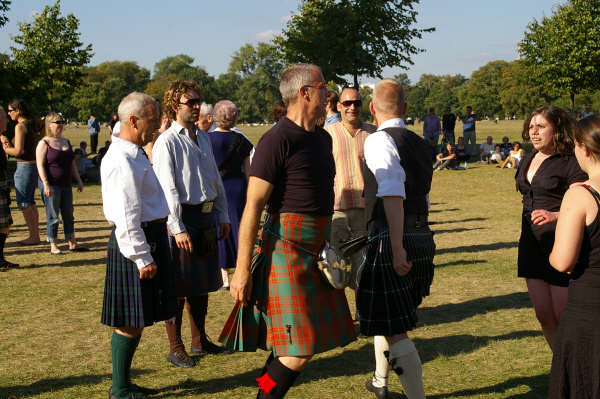This colour photograph, taken outdoors in what appears to be a large, expansive public park or the gardens of a stately home, features a broad field of short-cut, slightly yellowed grass with small grey patches. The background reveals a clear blue sky bordered by very tall, healthy trees and bushes, slightly turning brown with the changing season. The image captures numerous people gathered in several groups. In the foreground, a distinct group of men stands out, dressed in Scottish attire featuring navy blue and green and red plaid kilts, complemented by knee-high socks with ribbons. One man in this group appears to be in motion, as indicated by his slightly raised right knee and a hint of blur. This scene likely depicts a Scottish or Celtic gathering, with some men possibly preparing for a public performance, while others, including men in blue jeans and casual wear, mill about, chatting in the serene, verdant park.